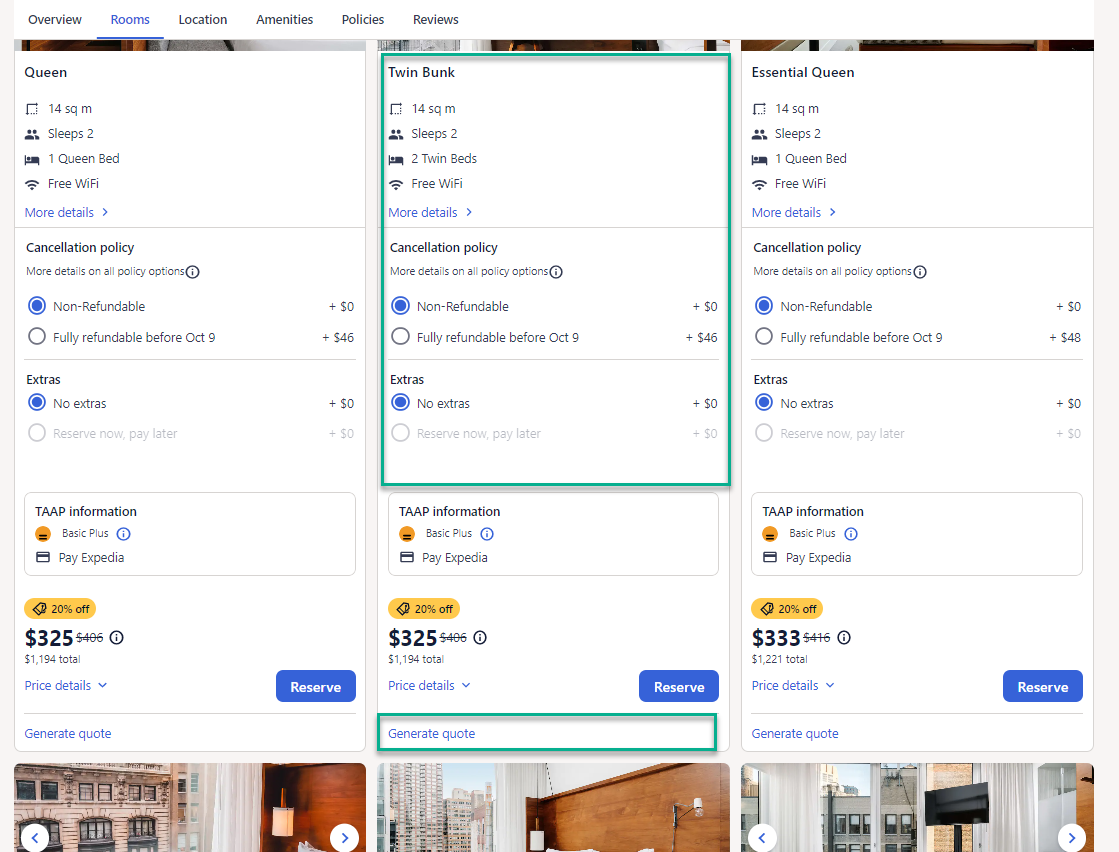The image resembles a travel website for booking hotel rooms, presenting a detailed interface for prospective guests. At the top left corner, there is a navigation bar with categories reading from left to right: Overview, Rooms, Location, Amenities, Policies, and Reviews. The 'Rooms' category is highlighted in blue, with a horizontal line underscoring it, indicating the current selection.

In the central panel of the page, three room options are displayed, each with accompanying details. On the left side, the first room is labeled "Queen" at the top left. The center room is marked as "Twin Bunk," and the rightmost room is identified as "Essential Queen." Each room listing includes an iconographic summary: all rooms measure 14 square meters, each accommodates up to two guests, and each room features specific bed types: the first has a queen bed, the second offers two twin bunk beds, and the third also has a queen bed. All rooms provide complimentary Wi-Fi.

Beneath the room descriptions, centrally located on the page, the cancellation policy is detailed. It offers two options: a non-refundable policy at no extra fee, and a fully refundable policy for an additional $46 charge.

The bottom section of the image displays the pricing for the rooms. The "Queen" and the "Twin Bunk" rooms are priced at $325 each, while the "Essential Queen" is slightly higher at $333.